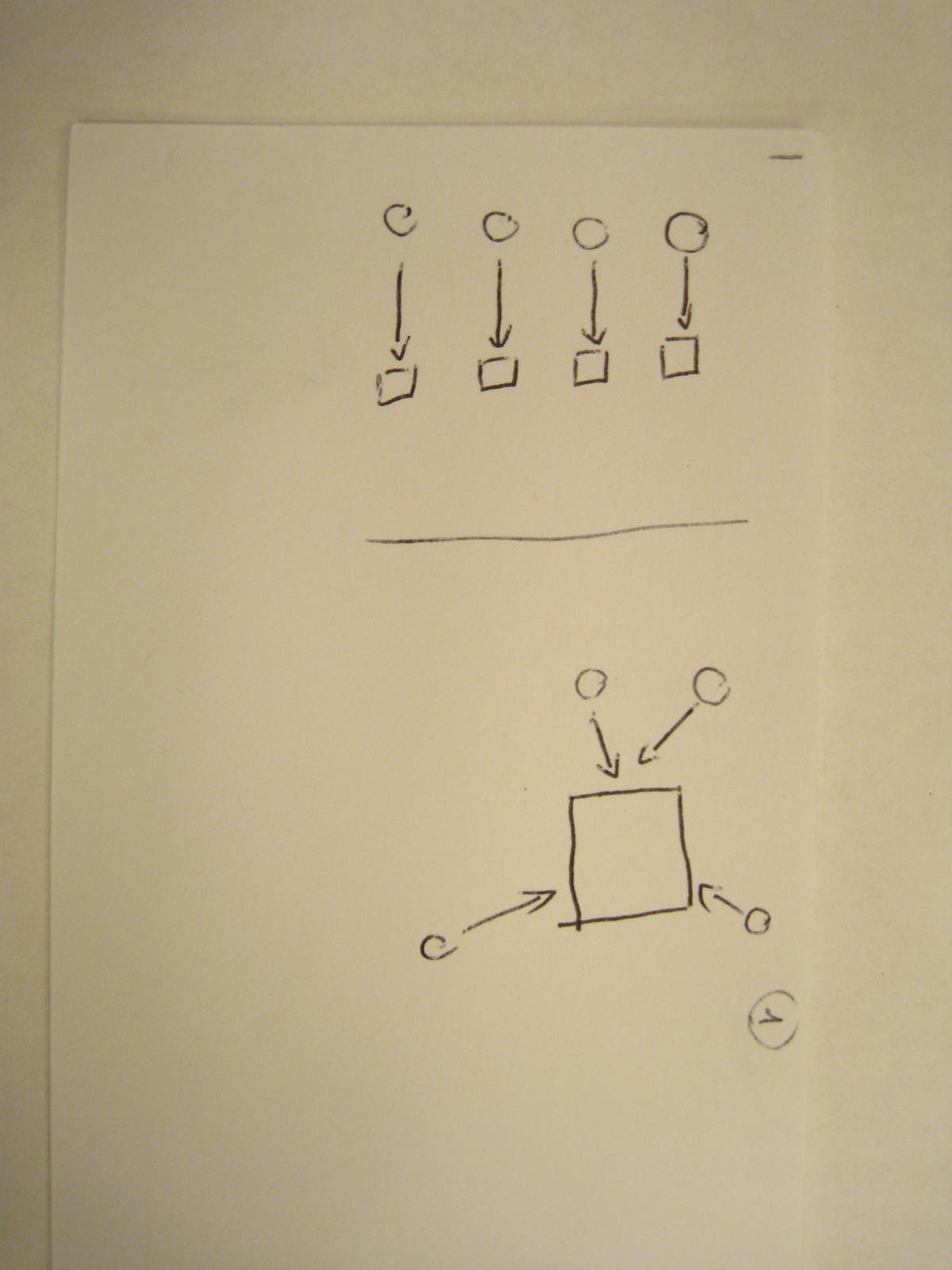The image presents a vertical sheet of paper, closely resembling the color of the off-white wall behind it, enhancing its subtle presence. The paper is affixed to the wall with a staple positioned in the top right corner, approximately 15% from the right edge and 5% from the left.

On this vertical sheet, a meticulous black ink sketch unfolds. About 10% from the top of the paper, there are four circles aligned horizontally, each positioned approximately 40% from the left edge. Arrows descend vertically from each of these circles, extending about 15% of the paper's height, connecting to small squares beneath each circle.

Further down the sheet, at around 40% of its height, a horizontal line spans the width, acting as a visual separator. Below this line, around the 50% mark, two additional circles are drawn. These circles feature similar downward arrows leading to a central, larger square. This larger square is also targeted by arrows originating from two more circles located in the lower right and lower left corners of the page.

This precise, symmetric arrangement of shapes and arrows creates a structured yet intriguing visual narrative on the otherwise understated, monochromatic background.